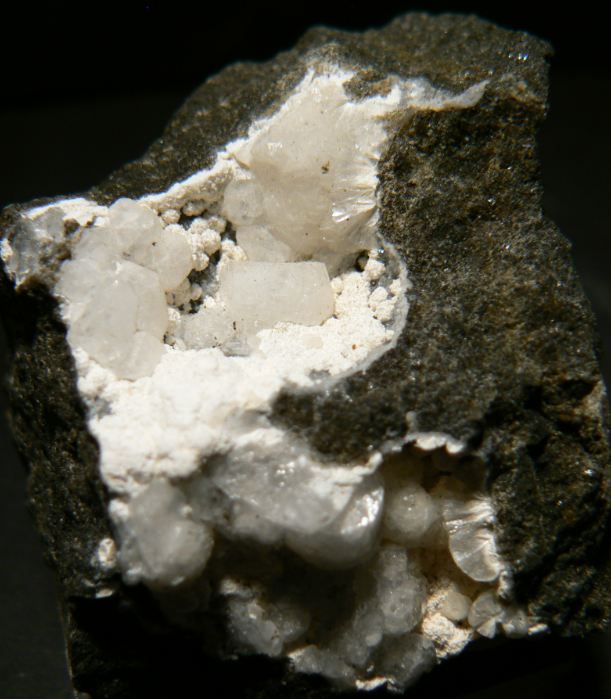This image features a close-up of a rock that has been split open to reveal its intricate interior. The exterior of the rock is a mix of gray, brown, and possibly green hues, resembling a conventional stone. The broken sections expose a striking white substance, which appears ceramic-like in hardness and structure. This inner layer is adorned with various crystals, some of which are shiny and form around the edges, while more densely packed, white crystals occupy the center. The top part of the inner section has a softer, almost glue-like appearance, overlaying what could be crystals in a more powdery form. The entire rock rests on a black background, providing high contrast that highlights the details of the crystalline formations and the textures within the rock.